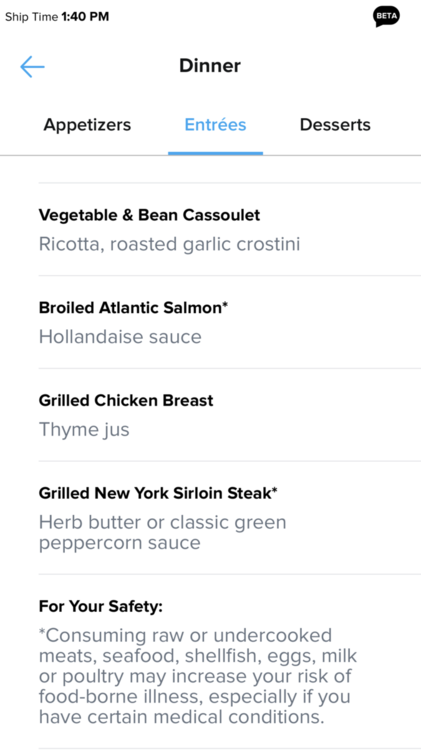**Screenshot of a Dinner Menu Interface**

At the top of the image, on a white background, "Ship Time 1:40 p.m." is displayed in black text. On the right side, there is a small black speech bubble with the word "Beta" in white text. Below this section, a blue arrow indicates the label "Dinner," followed by three categories: "Appetizers" in black, "Entrees" in blue with an underline, and "Desserts" in black. A thin gray line separates the categories.

The menu lists several items under each category:
1. **Vegetable and Bean Cassoulet**: Ricotta, roasted garlic, crostini.
2. **Broiled Atlantic Salmon**: Hollandaise sauce (an asterisk appears next to "Salmon").
3. **Grilled Chicken Breast**: Thyme juice.
4. **Grilled New York Sirloin Steak**: Herb butter or classic green peppercorn sauce (an asterisk appears after "Steak").

At the bottom, a note reads: "For your safety...," followed by an asterisk which leads to the cautionary statement: "Consuming raw or undercooked meats, seafoods, shellfish, eggs, milk, or poultry may increase your risk of foodborne illness, especially if you have certain medical conditions."